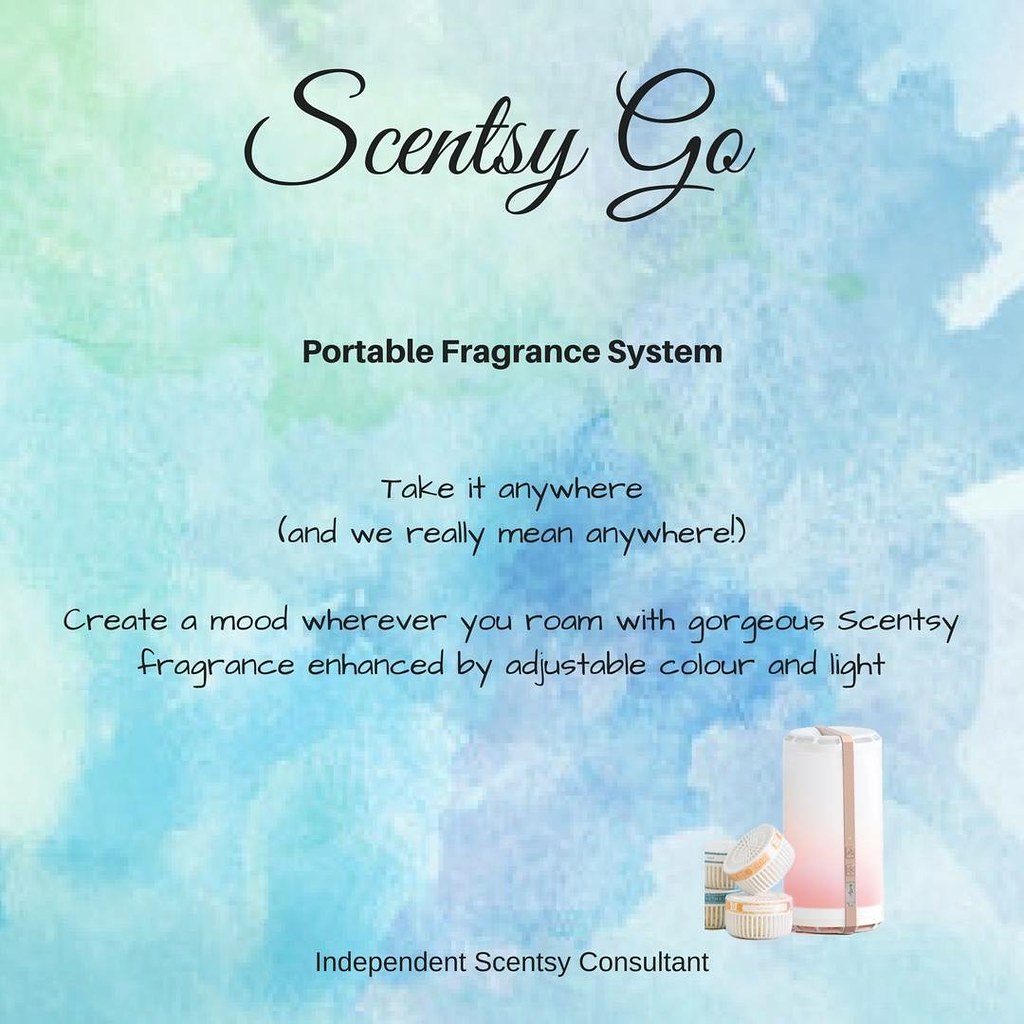The large square image is an advertisement with a visually appealing background, blending various shades of medium and light blue, with a touch of green in the upper left corner, giving it a mystical and cloudy sky appearance. At the top, the title "Scentsy Go" is written in cursive letters, followed by bold black text that states "Portable Fragrance System." Centered in the middle, the text continues in black, saying, "Take It Anywhere, and We Really Mean Anywhere," enclosed in parentheses. Further down, another line of centered black text reads, "Create a Mood Wherever You Roam with Gorgeous Scentsy Fragrance, Enhanced by Adjustable Color and Light." At the bottom, it mentions "Independent Scentsy Consultants." Positioned just above this line is an image depicting a cylindrical white and pink container, identified as the main product, alongside smaller round-shaped containers with lids, suggesting that these are the refillable scents making the system portable.